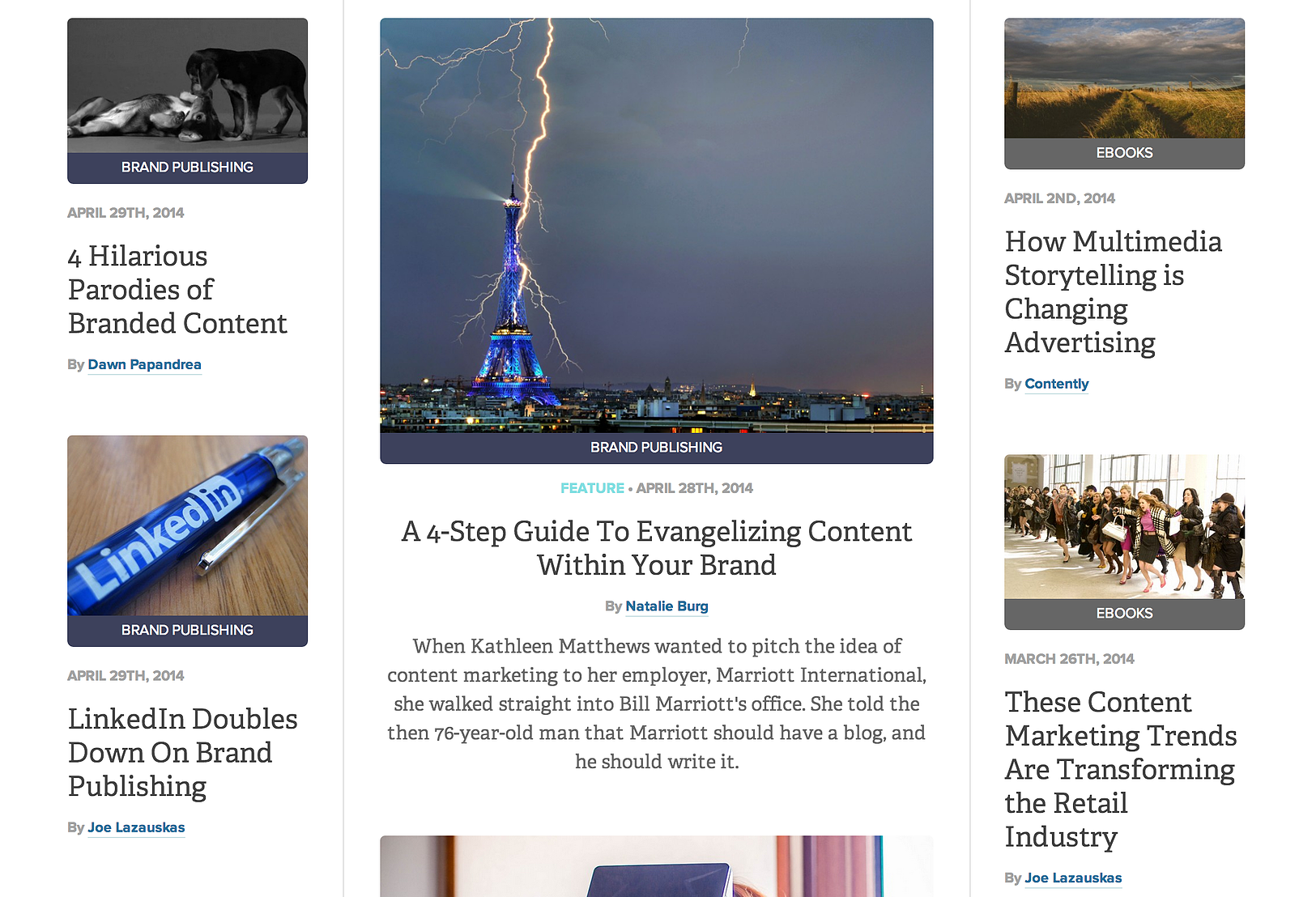In the center of the image, a dramatic dark night sky is captured, dominated by a massive lightning bolt striking down from above. This electrifying bolt hits the Eiffel Tower, which is illuminated in a striking blue color. Underneath this vivid scene, text reads: "Feature April 28th, 2014: A Four-Step Guide to Evangelizing Content Within Your Brand" by Natalie Berg. 

A narrative follows detailing how Kathleen Matthews proposed the concept of content marketing to her employer, Marriott International. She confidently walked into Bill Marriott's office and suggested that the then 76-year-old Marriott should start and personally write a blog for the company.

To the left of the main image, there are two smaller pictures. One is of two dogs, one black and one gray, with the caption "Four Hilarious Parodies of Branded Content" beneath it. Below the dogs, an image of a blue pen, emblazoned with the LinkedIn logo, is displayed alongside the text "LinkedIn Doubles Down on Brand Publishing."

In the upper right corner, an image showcases large, dramatic clouds above a long road flanked by yellow grass, captioned "How Multimedia Storytelling is Changing Advertising." Directly below this, there is an image of women standing on a white floor, all dressed in professional office attire, with the caption "These Content Marketing Trends are Transforming the Retail Industry."